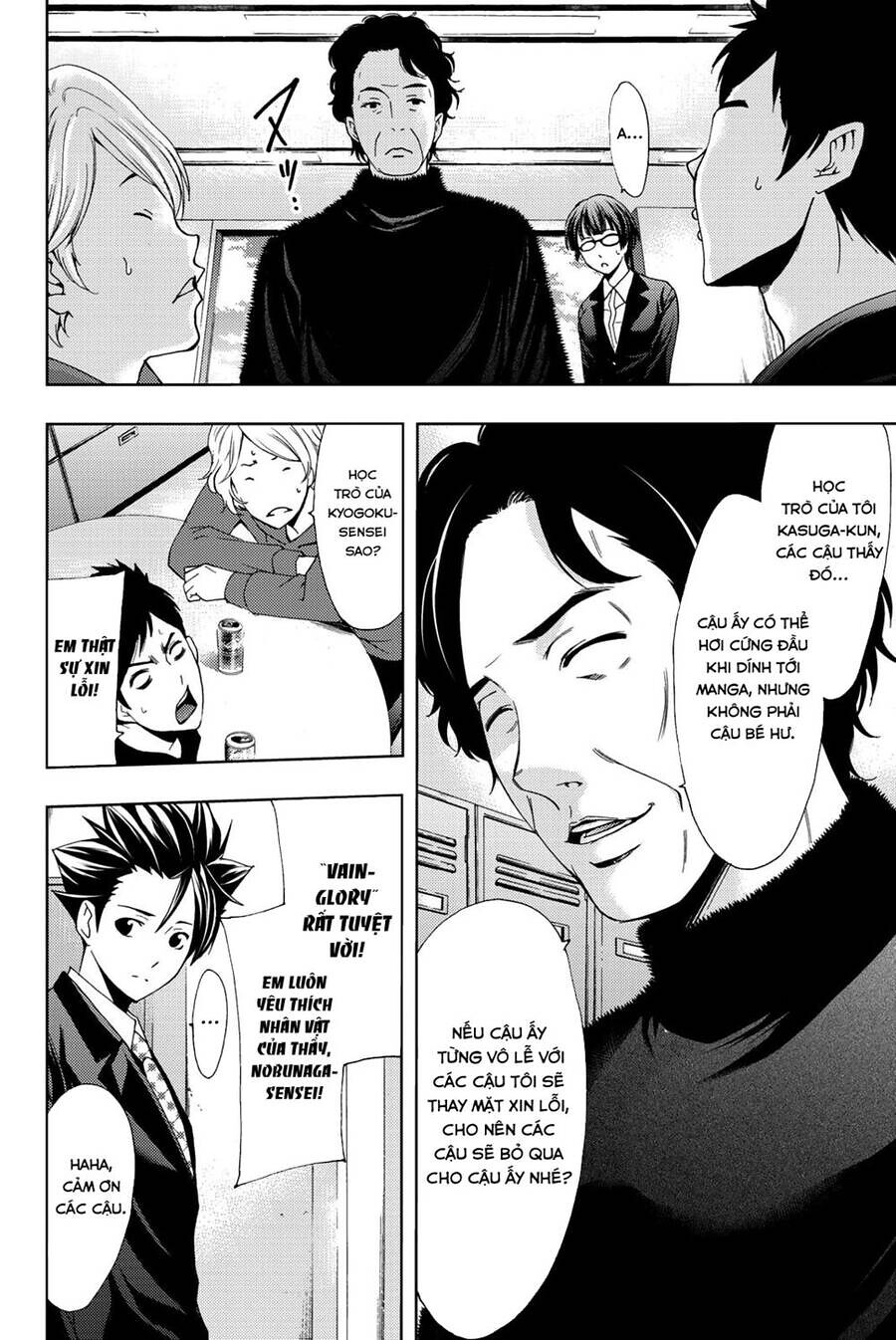The image depicts a four-panel, black-and-white comic that appears to be in Vietnamese, with some French language elements suggesting an Indochine influence. The layout consists of one long panel across the top and three smaller panels below, with the leftmost bottom panel split into two halves. The scene unfolds in a room with four characters: three with black hair and one blonde, whose genders are not clearly specified. The top panel shows all four people, where two characters in the forefront look anxiously at a stern-looking woman who has just entered. The subsequent panels likely capture their conversation, although the exact dialogue remains unreadable. The stern woman's expression softens to a smile in the bottom right panel, indicating a shift in the interaction. The entire comic reads from right to left, consistent with traditional manga formatting.